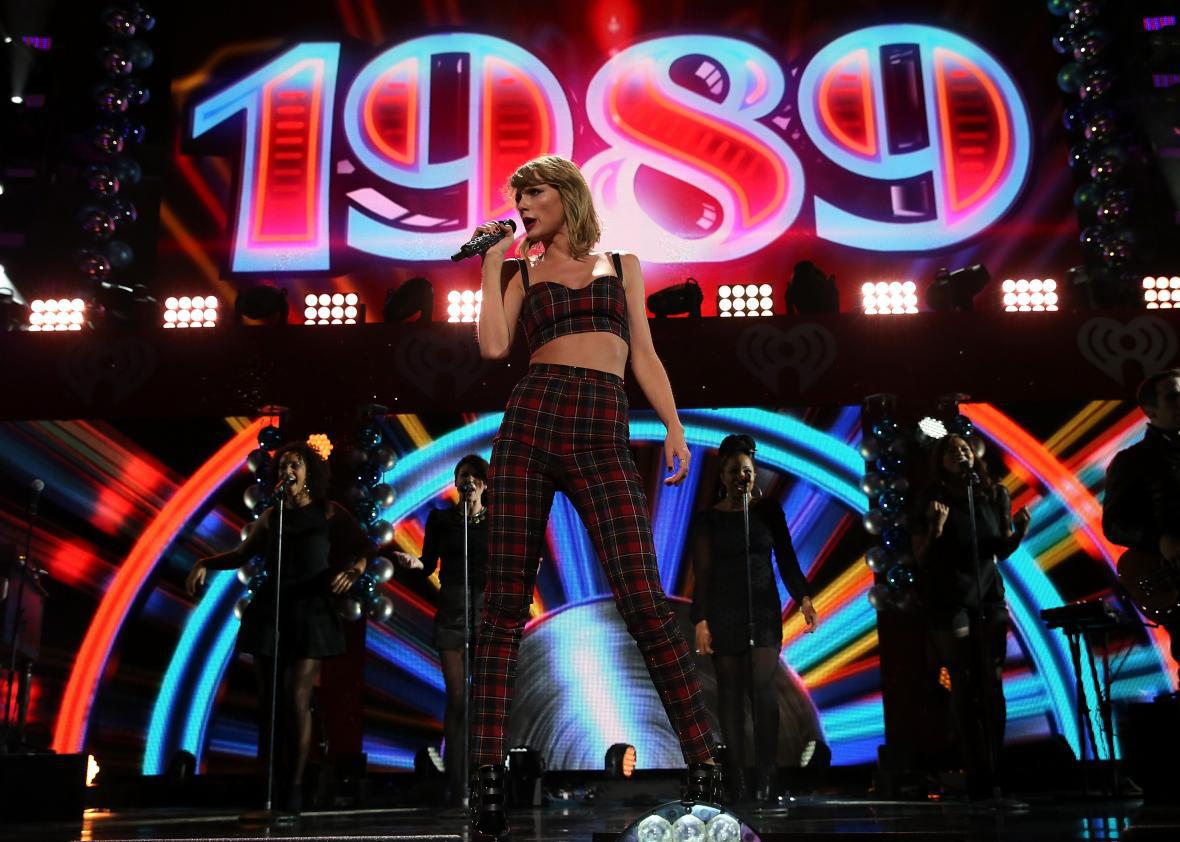The image captures Taylor Swift performing at an iHeartRadio event, standing center stage in the spotlight. She is holding a microphone with her right hand and looking to her right (our left). She sports a coordinated red and black plaid outfit consisting of high-rise tight pants and a midriff-baring top with thin spaghetti straps, exposing her abdomen. Behind her, five background singers are positioned to the right and left, dressed in all black and partially obscured by the stage’s lighting. The backdrop features a large "1989" illuminated in an old-school Broadway style, accompanied by circular neon-colored lights. There's also an iHeartRadio heart logo prominently displayed between the large "1989" sign and the colorful video screen below it. Although the image is zoomed in on Taylor, the intricate stage design and lighting emphasize the vibrant and energetic atmosphere of the night.